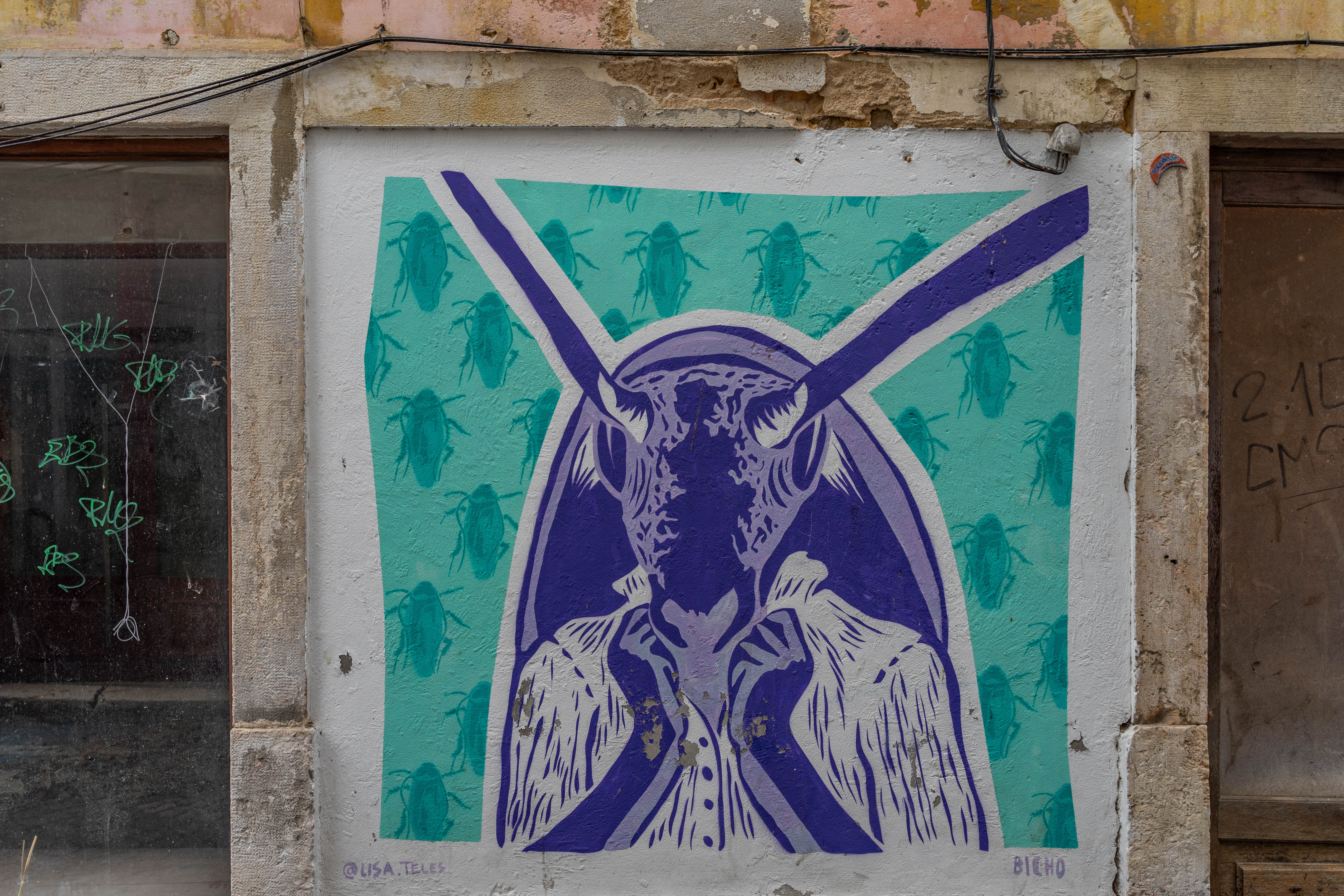This image showcases a detailed mural by the artist Blen Busa, located on the side of an old, crumbling building with stonework and chipped wood. The rustic and deteriorating industrial backdrop features graffiti tags, broken cement, and wires running across the scene. The focal point of the mural is a white-painted rectangular area with a turquoise background that displays a repeating pattern of darker turquoise cockroaches or beetles. At the center of this pattern is a surreal, half-bug, half-human character, adorned in a purple and white colonial-style military jacket with a purple-lined white frilly shirt. This character, which merges human arms and a bug-like face, adds a fantastical element to the mural. On either side of the mural, there are glass windows marked with graffiti, and additional writing, including 'CMC21E,' can be seen on the right side. The artwork is signed 'USA Tillis' and 'blend,' lending insight into the creative minds behind this compelling street art.